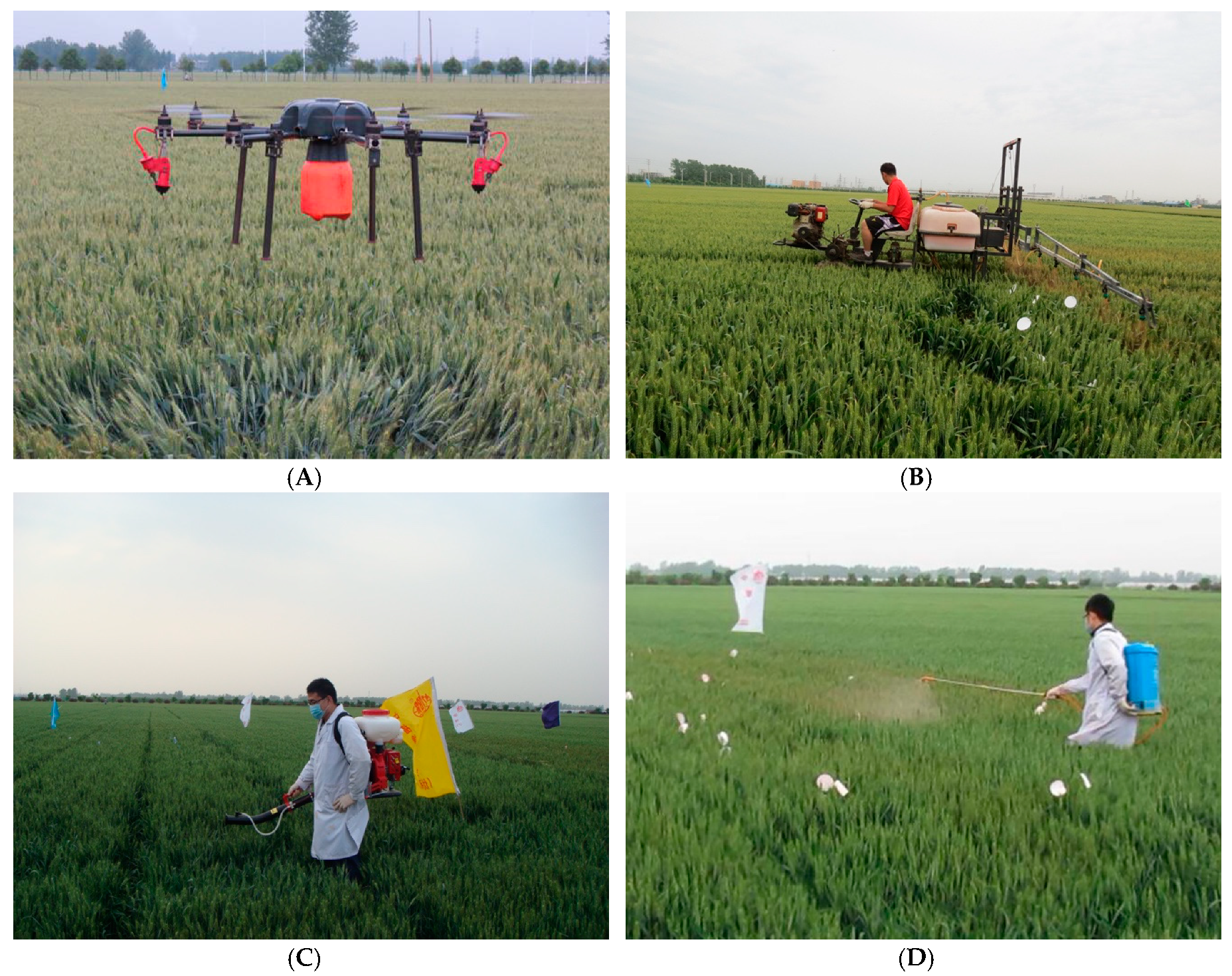The image is a compilation of four color photographs, each labeled with a black letter in parentheses: A, B, C, and D, depicting various methods of herbicide application in a sprawling field. 

- **Photo A (top left)**: Depicts a four-legged drone with orange tanks and propellers atop its arms, hovering above a grassy field with rows of trees in the distance under a hazy sky.
- **Photo B (top right)**: Shows a man in a red shirt and black shorts riding a motorized tractor equipped with a chemical tank and a broad spray arm, navigating the expansive field towards the left.
- **Photo C (bottom left)**: Features a person in a white lab coat, face mask, and a red and white tank structure on their back, using a short spray wand to apply herbicide. They are walking leftward in the field adorned with yellow and multicolored flags.
- **Photo D (bottom right)**: Illustrates another worker in a white coat with a blue tank on their back, facing left and spraying weeds in the grassy field.

The consistent themes of hazy skies and expansive fields reinforce the context of industrial-scale gardening or farming in each photograph.